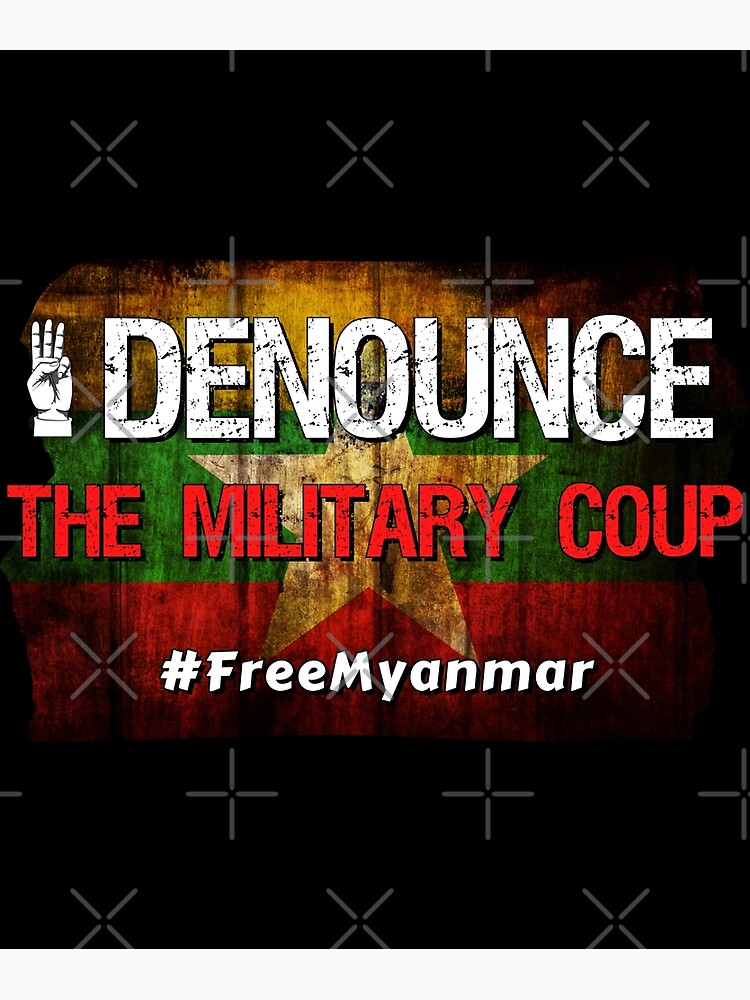The image showcases a bold graphic design with a predominantly black background interspersed with rows of alternating white or gray X's and plus signs that do not connect in the middle. Central to the design is the flag of Myanmar, characterized by its yellow top, green middle, and red bottom, with a prominent white star at its center. Superimposed on the flag is text advocating for political change. The text "Denounce" is written in gritty, bold white letters, next to a white hand making a three-finger salute. Below it, the phrase "the military coup" appears in bold red letters, followed by "#FreeMyanmar" in white. The graphic includes multiple white crosshairs suggesting a targeted focus on the message.